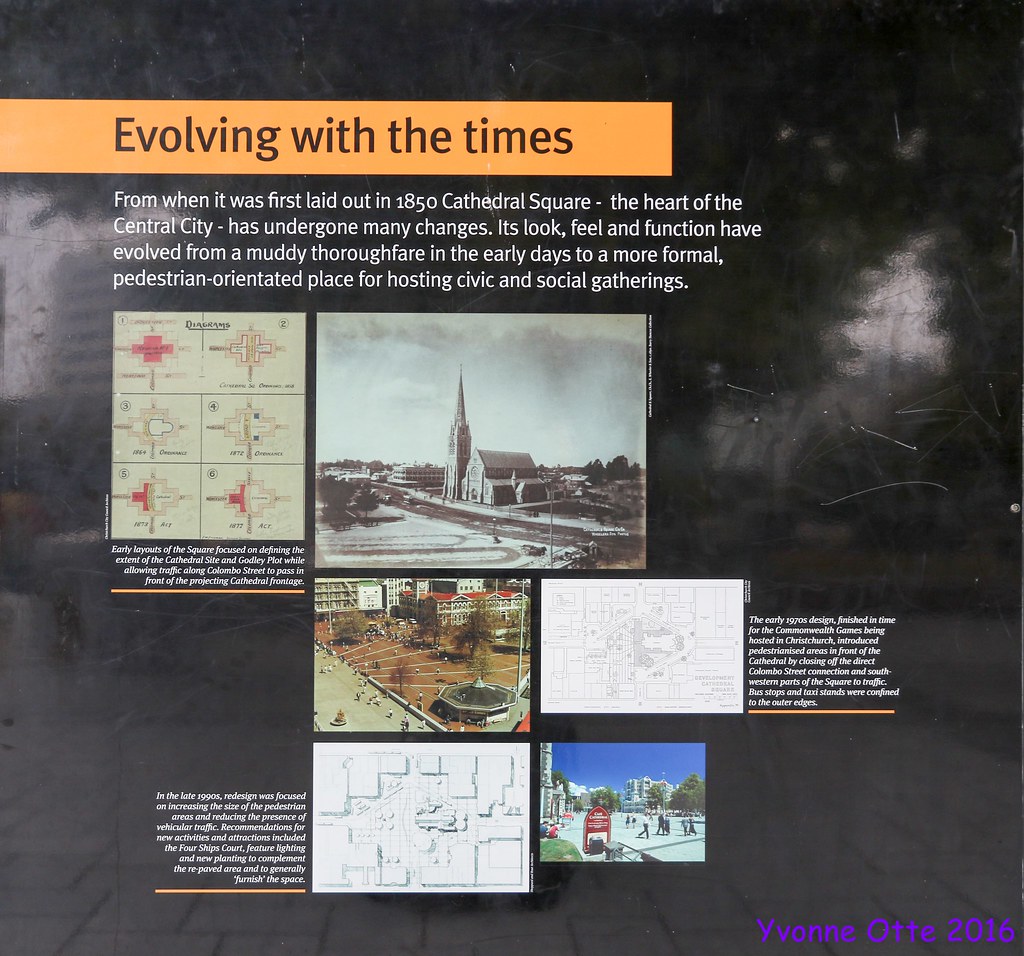The image features a smooth, dark black background, possibly resembling marble or slate. Prominently displayed at the top left is an orange rectangular banner with black lettering that reads "Evolving with the Times." Beneath this, in smaller white text, it states: "From when it was first laid out in 1850, Cathedral Square, the heart of the central city, has undergone many changes. Its look, feel, and function have evolved from a muddy thoroughfare in the early days to a more formal, pedestrian-oriented place for hosting civic and social gatherings." Below the textual information, there is a masonry-like layout of images and schematics, providing a visual timeline that captures the evolution of Cathedral Square. Starting from a black and white photo of the original cathedral, transitioning to colored photos of the present-day plaza, and interspersed with various schematics and maps, these visuals highlight the square’s historical transformation. In the bottom right corner, the name "Yvonne Otte, 2016" is written in blue, adding a subtle signature to the composition.